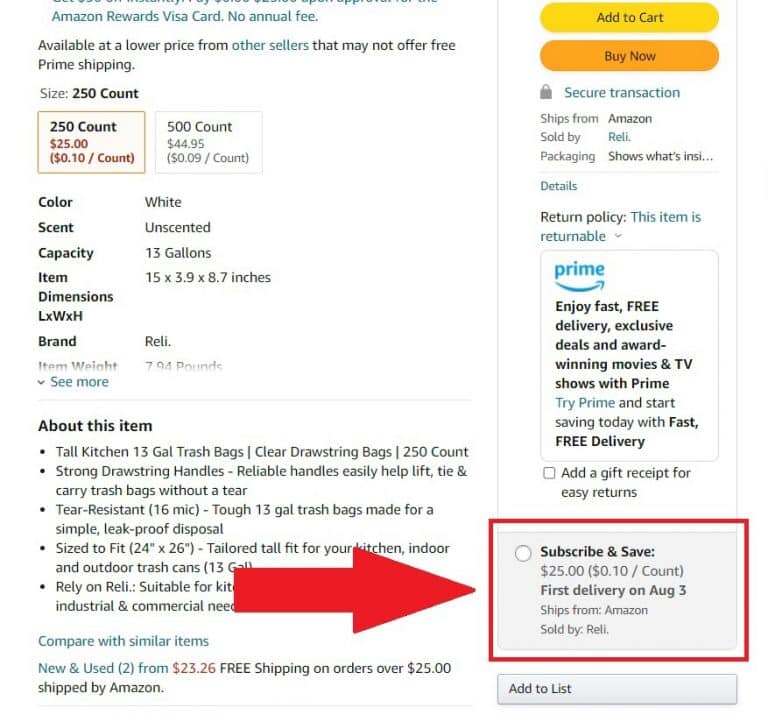The image appears to be a screenshot from an Amazon Prime product page. In the top right corner, there is a prominent "Add to Cart" button in black, set on a yellow, oval-shaped rectangle. Just below this is the "Buy Now" button in orange, similarly shaped. Under these buttons, the text "Secure transaction" is visible, followed by "Ships from Amazon" and "Sold by Raleigh." The note "Packaging shows what's inside" appears, although the word "inside" is partially cut off.

Continuing downwards on the middle right side, it states "Return policy: This item is returnable." Below this, there is a square section with the Prime logo that reads, "Enjoy fast, free delivery, exclusive deals, and award-winning movies and TV shows with Prime."

Near the bottom right, a red rectangle has been drawn, highlighting the "Subscribe & Save" section. Within this highlighted area, it mentions "$25. First delivery on August 3rd." Additionally, a red arrow at the bottom middle points towards this area for emphasis.

At the top left of the image, specific product details are provided: "250 count, 10 cents per count, color: white, scent: unscented, capacity: 13 gallons." Further down in the center, there is a section labeled "About this item," offering more detailed product information.